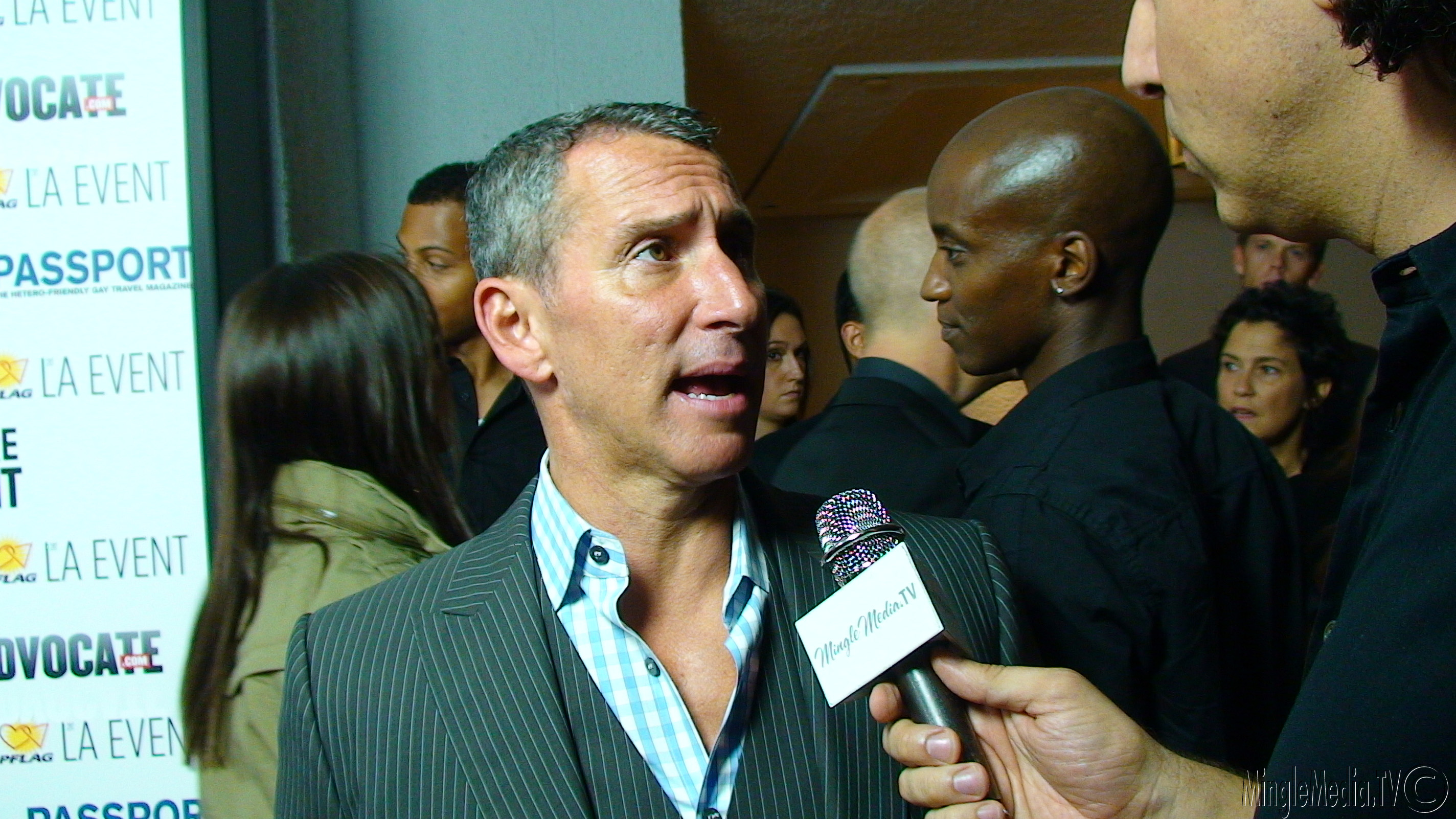In this horizontally aligned rectangular photo, a man is being interviewed at an event. He has short salt-and-pepper hair and is wearing a thin pinstripe black and white suit over a white and blue plaid button-down shirt, which is unbuttoned at the top. His mouth is open, revealing his bottom teeth, and he has either tan or slightly darker skin, possibly in his 40s or 50s. We see the right side and front of his face as he speaks into a microphone held by a taller person on the right side of the image. The microphone has a distinct white triangular logo with the words "Mingle Media TV". The interviewer, a white male with dark hair, is dressed in a navy blue or black button-down shirt, though only the left lower part of his face and neck are visible. In the background, a crowd of people are mingling, engaged in conversation, while a wall on the left side displays repeated texts including "LA event", "events", and "advocate".